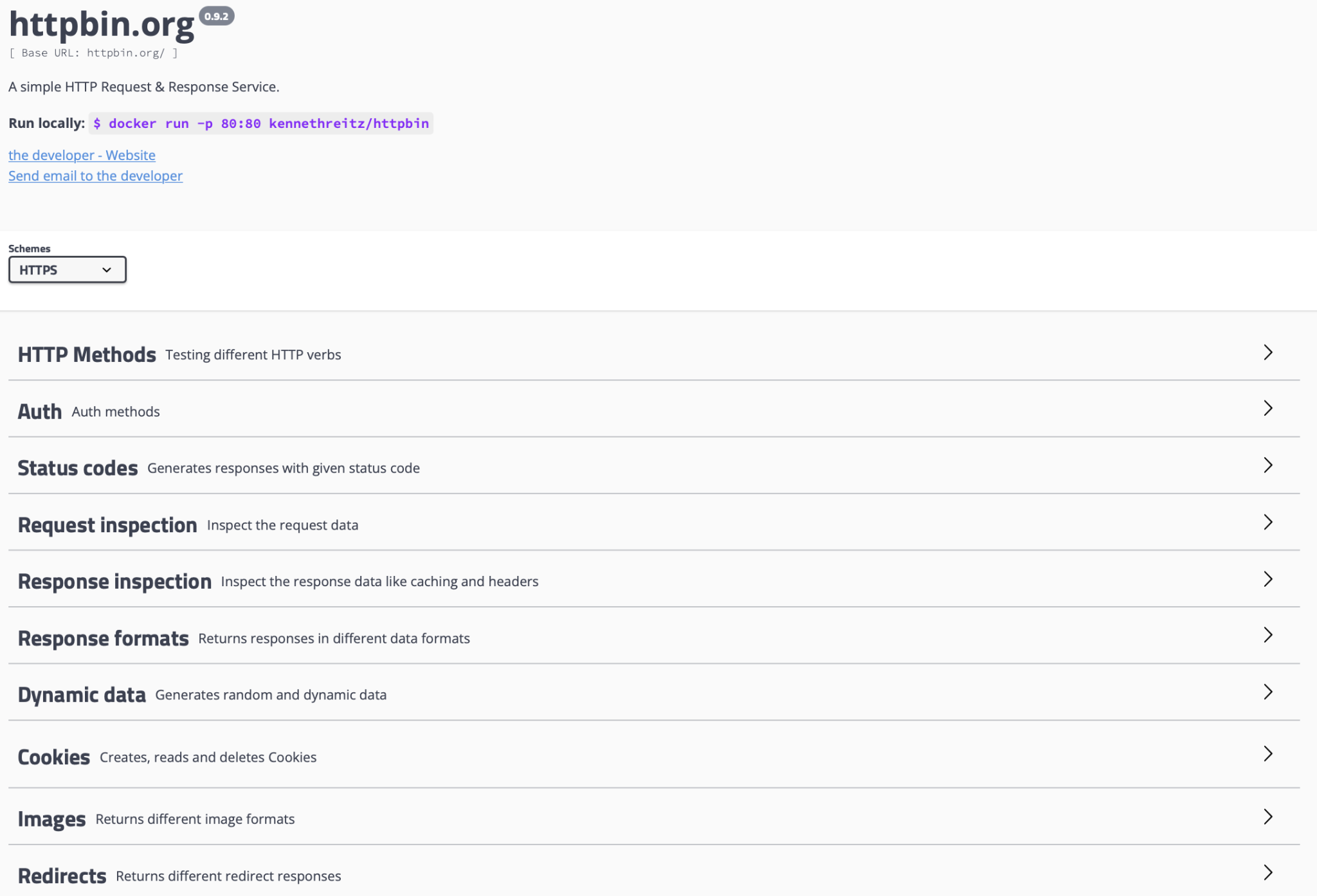The image is a computer screenshot with a predominantly light gray background and a horizontal rectangular format. In the upper left corner, the text "httpbin.org" is prominently displayed in bold black font, accompanied by a subheading that reads "A simple HTTP request & response service. Run locally." Directly beneath this, a line of code is shown, starting with a purple dollar sign ($) followed by "docker run" and additional technical details that are not fully discernible. 

Highlighted in blue are two clickable links: "The Developer Website" and "Send Email to the Developer." Below these links, there is a section titled "Schemes," containing a dropdown box with "HTTPS" displayed and an adjacent down arrow indicating more options.

The main content of the screenshot features a list of approximately ten clickable lines, each providing further options for interaction. The first line, in bold, reads "HTTP Methods," followed by a description "Testing different HTTP verbs" and a right-pointing arrow on the far right. Subsequent lines are similarly structured, including "Auth" (short for authentication methods), and "Status Codes" with the description "Generates responses with given status code," each ending with a right-pointing arrow to indicate additional information accessible upon clicking.

Overall, the screenshot depicts a well-organized user interface designed for developers to interact with and test HTTP requests, authentication methods, and status codes, among other functionalities.